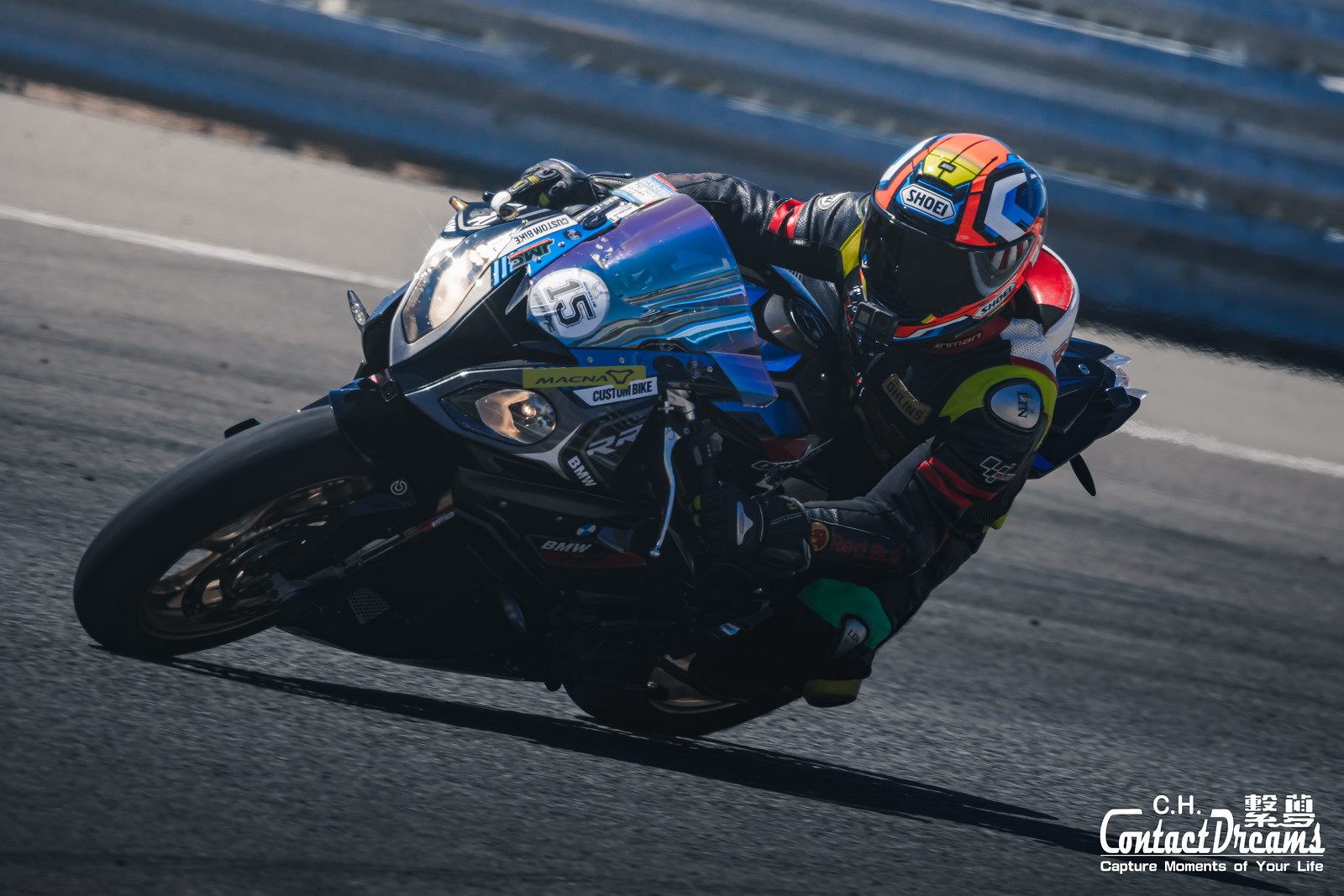A vibrant image captures a motorcyclist in the midst of a sharp left turn on a motorcycle track. The rider, adorned with a multi-colored helmet featuring hues of orange, yellow, blue, black, and white, is deeply leaning to the left, showcasing an intense moment in the race. His dynamically colored safety gear—yellow, black, red, green, and blue—adds to the visual excitement. The blue motorbike, accented with patches of yellow, purple, and gray, is angled sharply as it navigates the curve of the track, with the number 15 prominently displayed on the front windshield. The backdrop features a gray track, shoulder, and a metal girdered fence, neatly dividing the image. Centered in the frame, the photograph also includes a white textual overlay at the bottom half, reading "CH contact dreams. Capture moments of your life,” against the gray asphalt, emphasizing the thrilling capture of a high-speed moment.